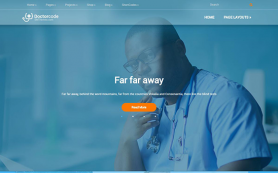This image appears to be a small, likely mock-up, screenshot of a medical website. The central figure in the image is an African-American male, seemingly in his early 40s, dressed in blue doctor scrubs, wearing spectacles, and a stethoscope draped around his neck. He is slightly turned to his right with his right index finger resting thoughtfully on his chin, a gesture directed towards the camera. 

The top of the image features a blue navigation bar with an indistinct logo displaying a stethoscope, alongside a home button and other unreadable icons. Below this bar, white text with the phrase "Far, far away" stands out on a darkened overlay, designed to enhance readability. Further down, there is a line of barely legible small white text, followed by an orange call-to-action button shaped like a capsule with white text that is difficult to decipher.

The entire screenshot measures only about two inches in width and one-and-a-half inches in height on the viewer's screen, making detailed examination a challenge. The blurred background hints at a medical setting, possibly an examination or operating room, although the exact nature of the environment remains unclear due to the image's tiny size and low resolution.